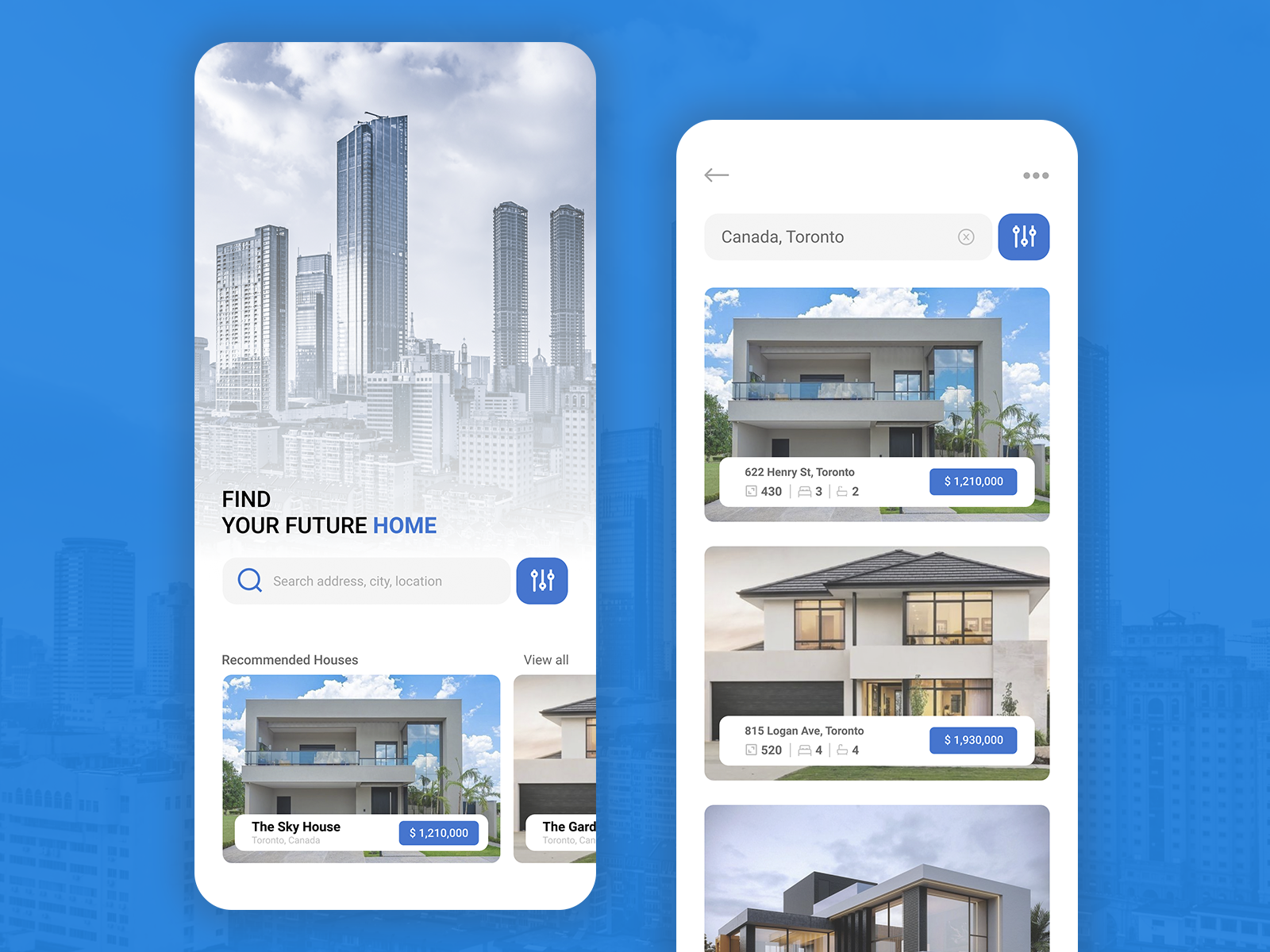In this detailed image, two screenshots of a real estate app are displayed side by side against a backdrop with a blue filter overlaying a cityscape photo. On the left screen, a promotional banner featuring tall buildings is accompanied by the text "Find your future home." Below the banner, a search bar is pre-filled with "Search address, city, location," followed by a list labeled "Recommended houses," featuring properties like "The Sky House" and a partially visible "The Garden."

On the right screen, the search bar displays "Canada, Toronto," and lists search results. The first result is "The Sky House," priced at $1,210,000, matching the left screen's recommendation. The second result, priced at $1,930,000, appears to correspond to the truncated second recommendation on the left screen, though its full name isn't visible. A third image appears at the bottom but is cut off, leaving its details obscured. The overall layout aims to provide users with an intuitive and appealing interface for discovering potential homes.